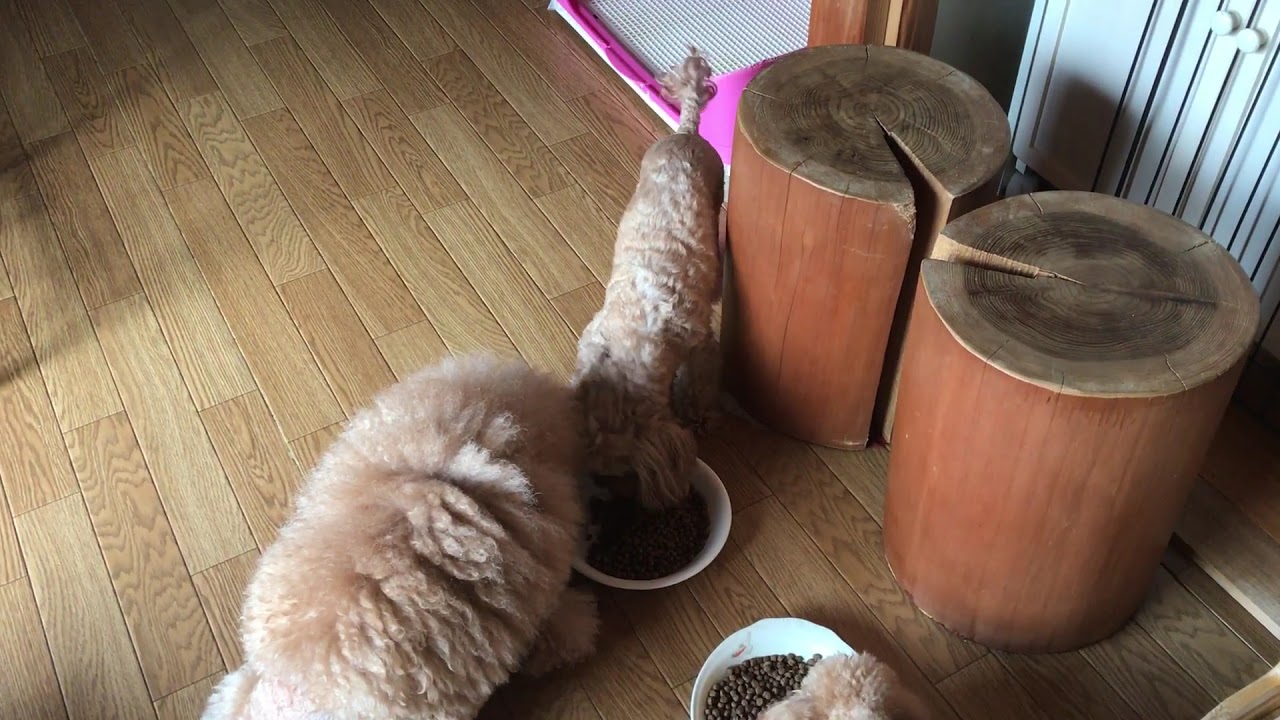The horizontally aligned rectangular photo depicts an indoor scene, likely in a kitchen or pet feeding area, set in the middle of the day. On a light pine-colored wooden tile floor, two round white bowls filled with dog food pellets are placed side by side. A small, fluffy dog with beige, light brown hair and another smaller dog with short brown hair, identifiable by its styled tail, are centrally positioned, sharing one of the bowls. At the very bottom of the image, only the head of a third dog, also light brown, is visible as it eats from the other bowl. In the background, two medium-brown wooden barrels, each marked by an ax cut, stand vertically. Behind them, a white wall can be seen. The overall image is dominated by shades of brown, white, and tan.